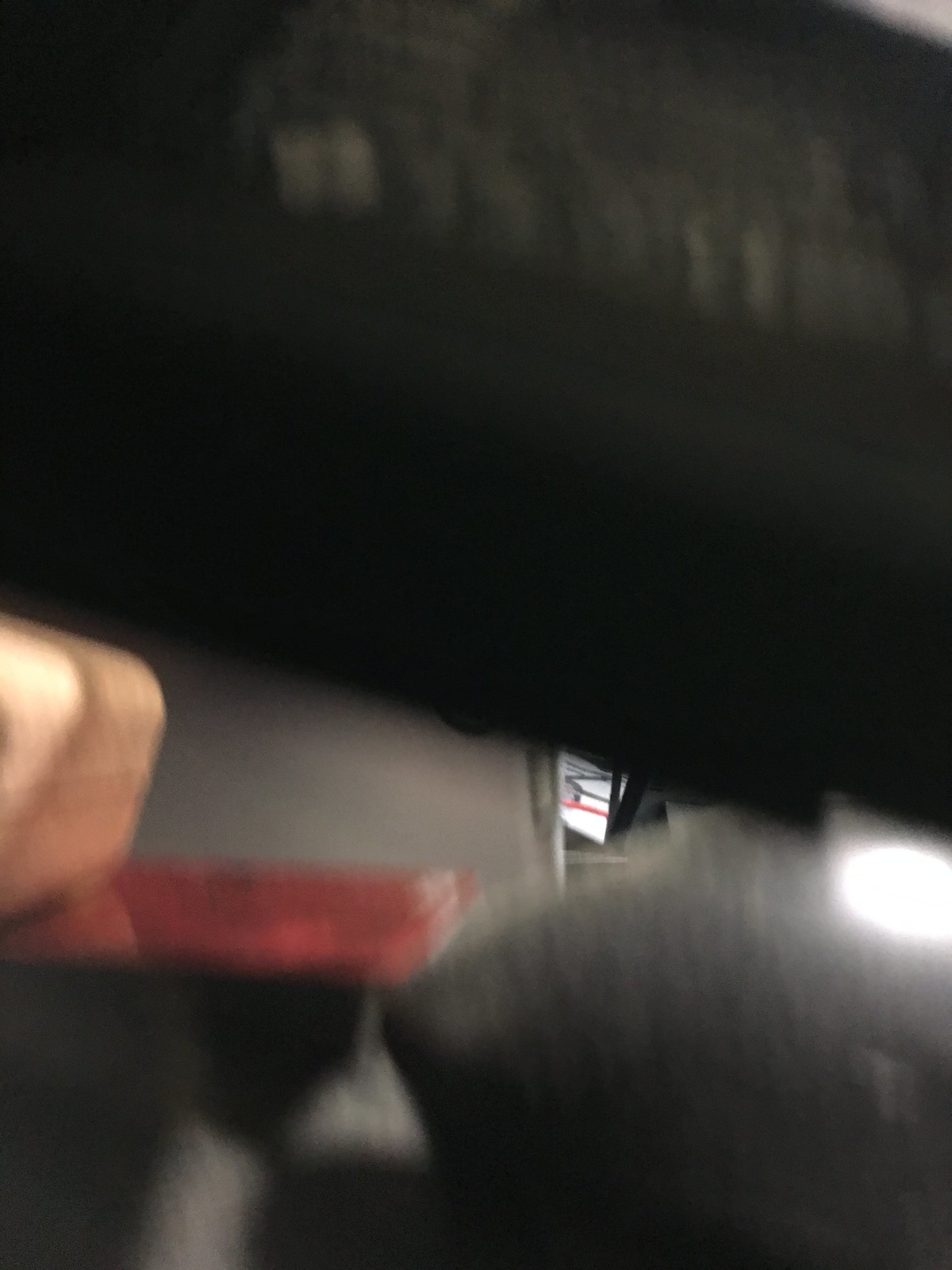This image is very blurry and dark, with areas of overexposure that obscure its contents. The top portion of the image contains a dark object, possibly black and cotton-like, which is indistinct due to the blurriness. Below this, towards the left, is a golden or beige square intersecting the frame, resembling a person's hand, though not clearly identifiable. Adjacent to it, a red, shiny rectangle is partially visible with a gray background behind it. A reflective black surface occupies the bottom right corner, featuring a bright, oval-shaped white light spot. The middle part of the image shows some letters, though their meaning is unclear, adding to the overall ambiguity and indistinct nature of the scene.